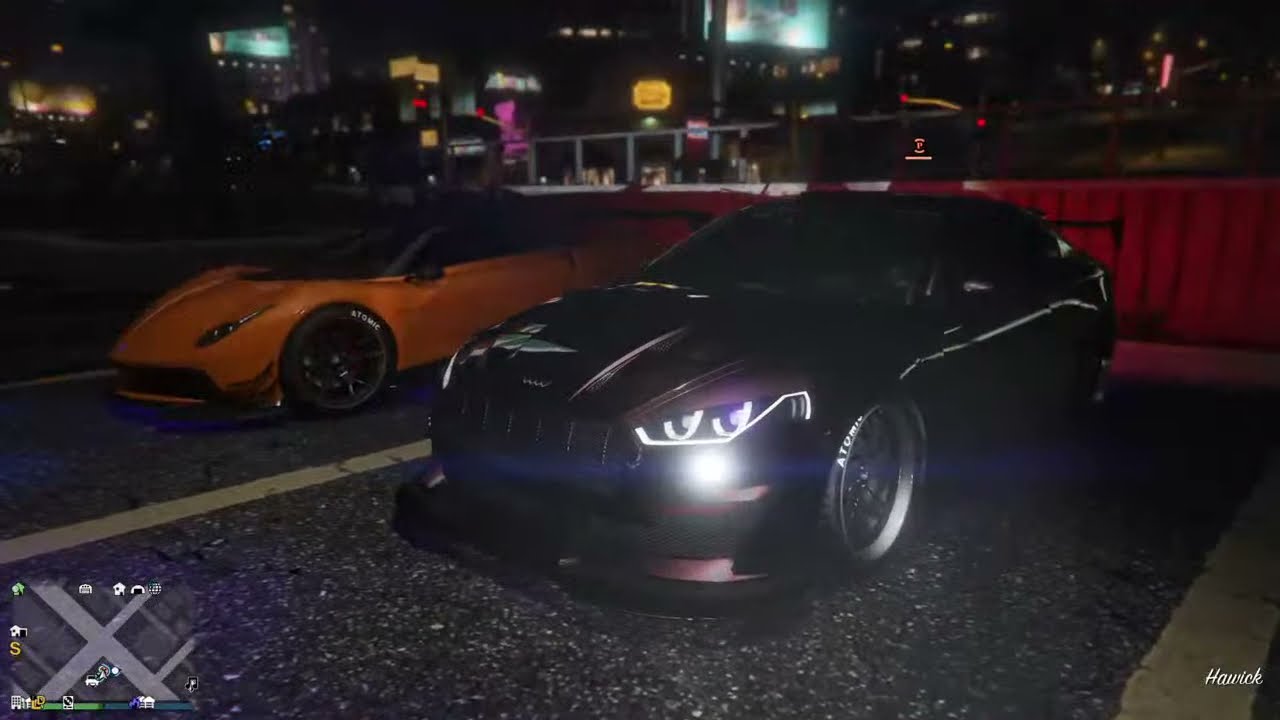The image showcases a nighttime scene reminiscent of a video game, showing a parking lot illuminated against a vibrant city skyline. In the parking lot, there are two prominently parked sports cars. The car on the far left is a striking orange, resembling a high-performance model like a Corvette or Camaro, featuring black rims and thin-walled tires with "atomic" written in white. It also sports a black top and a sleek spoiler. To its right is a dark-colored sports car, potentially a deep plum or dark gray shade, also highlighted by its headlights being on. This vehicle, possibly an Audi, has a two-door design, a vertical grille, black wheels, and "atomic" branded tires, with its features suggesting high maneuverability for cornering. The scene, framed in a rectangular format approximately six inches wide and four inches tall, includes additional elements like a small map of the game in the lower left corner and the word "Hawick" written in white cursive on the lower right. A red raised area, suggestive of a curtain, along with city lights, a digital billboard, a railing, and street lights, forms the backdrop, enhancing the urban aesthetic.